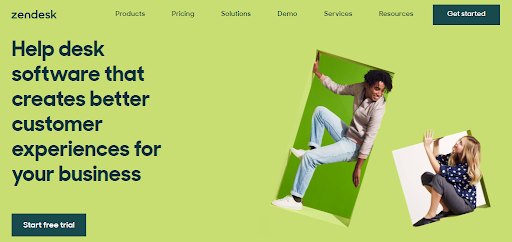This image is a screenshot of the Zendesk website. The background is a striking lime green. At the top of the site, the word "Zendesk" is prominently displayed in blue. Adjacent to this, on the right, is a navigation bar with the following options: Product, Pricing, Solutions, Demo, Services, and Resources. There is also a prominent blue button labeled "Get Started."

On the left side of the screenshot, the text "Helpdesk software that creates better customer experiences for your business" is prominently featured, followed by a "Start Free Trial" button below it.

To the right, there is an illustration of a man with brown skin, black hair, wearing a beige shirt, blue jeans, and white shoes. He is leaning into a window cutout with a dark green background, looking down at a woman. The woman, with white skin, is depicted in a smaller white window below. She has blonde hair and is dressed in a blue shirt with white polka dots, gray pants that end at her calves, and black shoes. She is gazing up at the man.